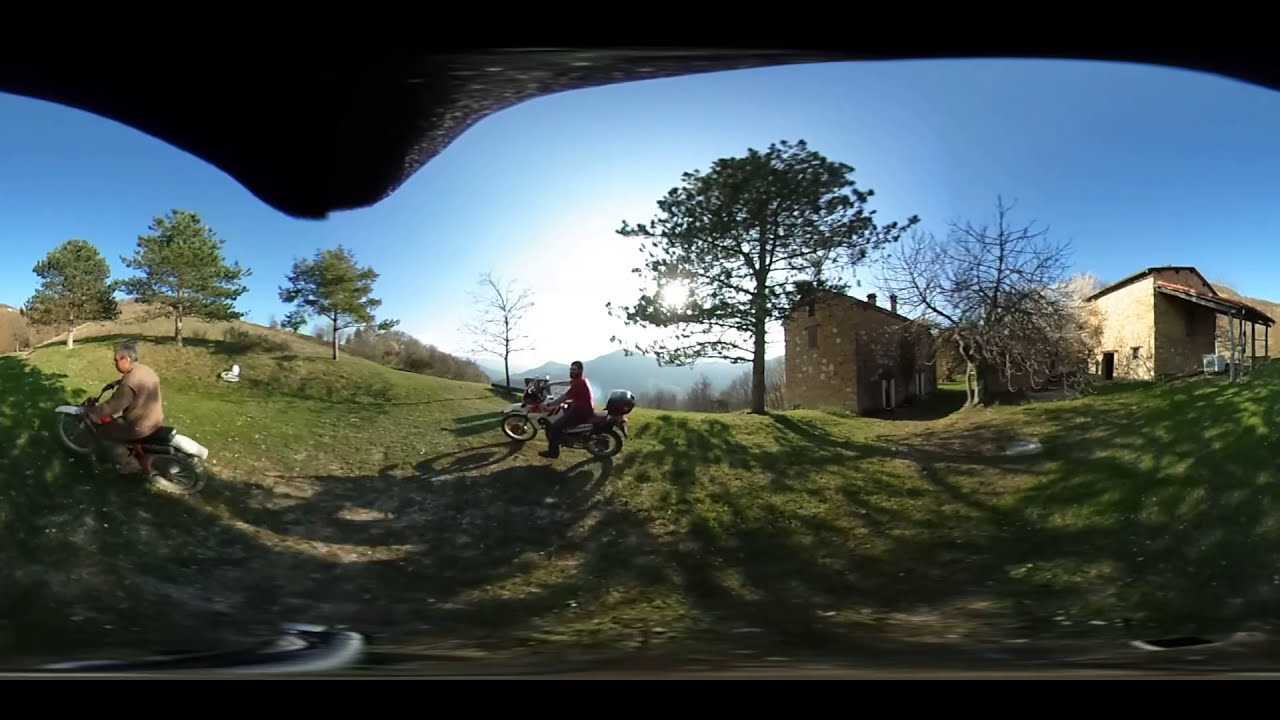The image depicts a panoramic view of two older men, possibly in their 40s or 50s, riding motorcycles on a grassy area, which seems to be expansive countryside. The motorcycle closest to the center, slightly to the left, is ridden by a man in a red shirt, while the man in a brown shirt rides on the far left. Both motorcycles are colored in white, black, and red. The background features several key elements: to the right of the centered rider is a tree next to a tan brick house with a red awning, followed by another tree in the middle and another similar house further right. Above the motorcyclist on the left are three trees on a gentle hill. The entire scene is divided horizontally; the lower half is lush green grass, and the upper half is a blue sky. The horizon reveals some distant mountains, adding to the scenic, open-air atmosphere, despite an unusual suggestion of being inside a cave-like structure with an arching ceiling, noted for the distorted panoramic effect. Nearby buildings on the hillside, appearing as stone-made storage sheds or older derelict structures, further accentuate the rural, relaxed vibe of the scene. Trees with green leaves and brown trunks are scattered throughout, emphasizing the natural surroundings. The photo captures a joyous moment, perhaps in someone's expansive backyard, with the individuals enjoying a carefree ride on their vehicles.